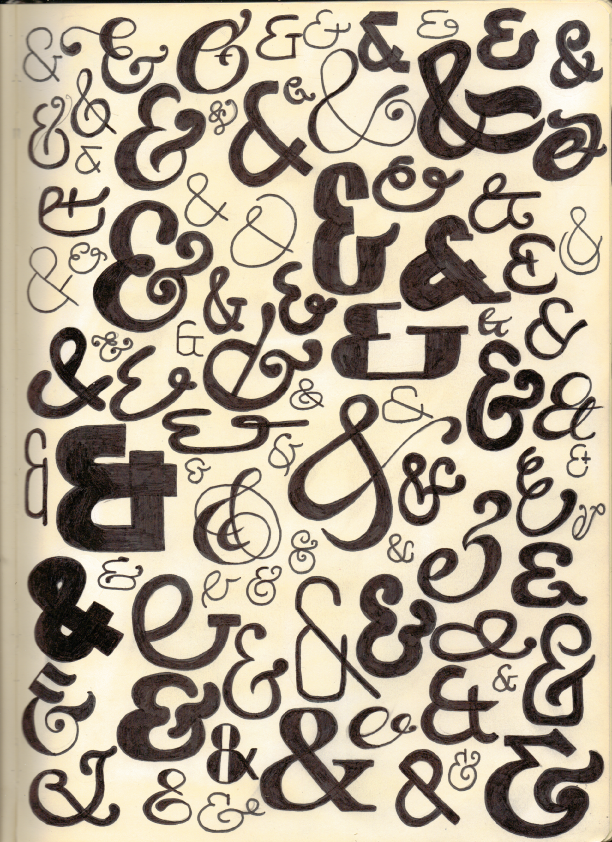This vertical rectangular image is a piece of art featuring an off-white or ivory-colored background that resembles paper. The artwork showcases dozens of black ampersands, varying in size, thickness, and font style. These ampersands are meticulously drawn with a felt pen, demonstrating a range of designs from straight to more ornate. They are scattered across the page in an organized yet chaotic manner, creating an intricate pattern of repetitive symbols. The visual effect is striking, with each ampersand contributing to the overall complexity and texture of the piece.